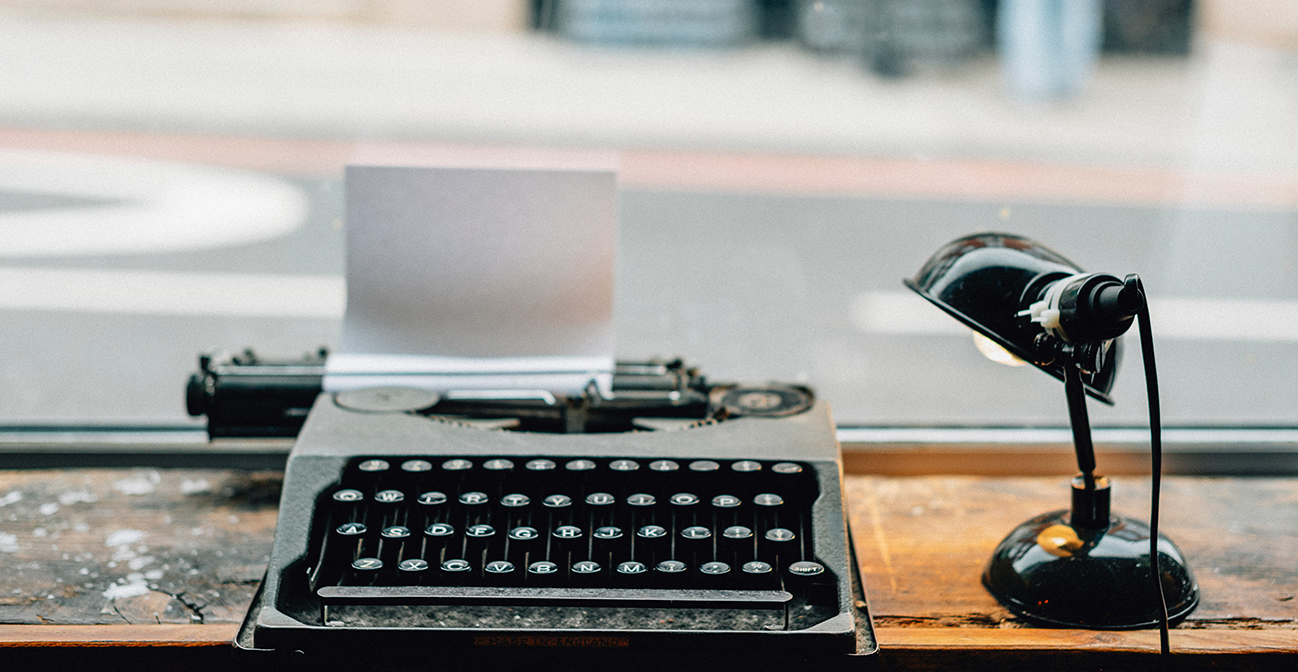This colored indoor photograph captures a vintage scene with an array of antique objects. The focal point is an old-style typewriter, gray or black, positioned on a worn wooden desk or table that features paint splatters, cracks, and signs of age. The typewriter, which may date back to the 1950s or 60s, has round keys and a movable carriage that is slightly shifted to the left. A sheet of white paper is inserted into the carriage. To the right of the typewriter stands a shiny black metal desk lamp, approximately 12 inches tall, with a visible light bulb and power cord. Notably, the lamp has been repaired with two zip ties. The lamp is on, illuminating the right side of the typewriter. The background is blurry but suggests a street scene beyond a window, possibly indicating the setting is in a coffee house. There are no other objects, images, or text in the foreground.